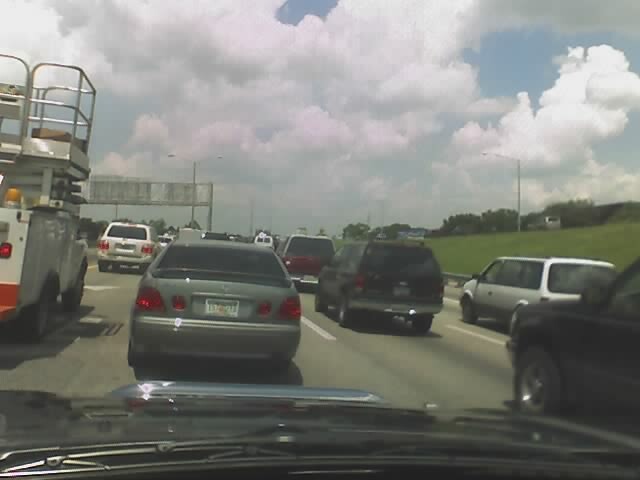Captured from a dash cam, this photograph reveals a bustling highway scene observed from inside a car, likely amidst traffic. Large, puffy cumulus clouds dominate the sky, casting shadows on a mostly sunny day with hints of a dirty blue sky peeking through. The highway is crowded with vehicles, featuring several lanes filled with cars all moving away from the camera's vantage point. Prominently, a gray sedan is visible directly in front, flanked by a black sedan to the right. In the upper left, a utility vehicle equipped with a cherry picker stands ready to service power lines or fiber cables. Street lights, power lines, and gray poles holding interstate signs are seen sporadically in the background. On the roadside, green grass grows on an incline, and trees are visible far off into the distance. The overall scene captures a typical, busy day on the interstate, emphasizing the heavy traffic and detailed surroundings.